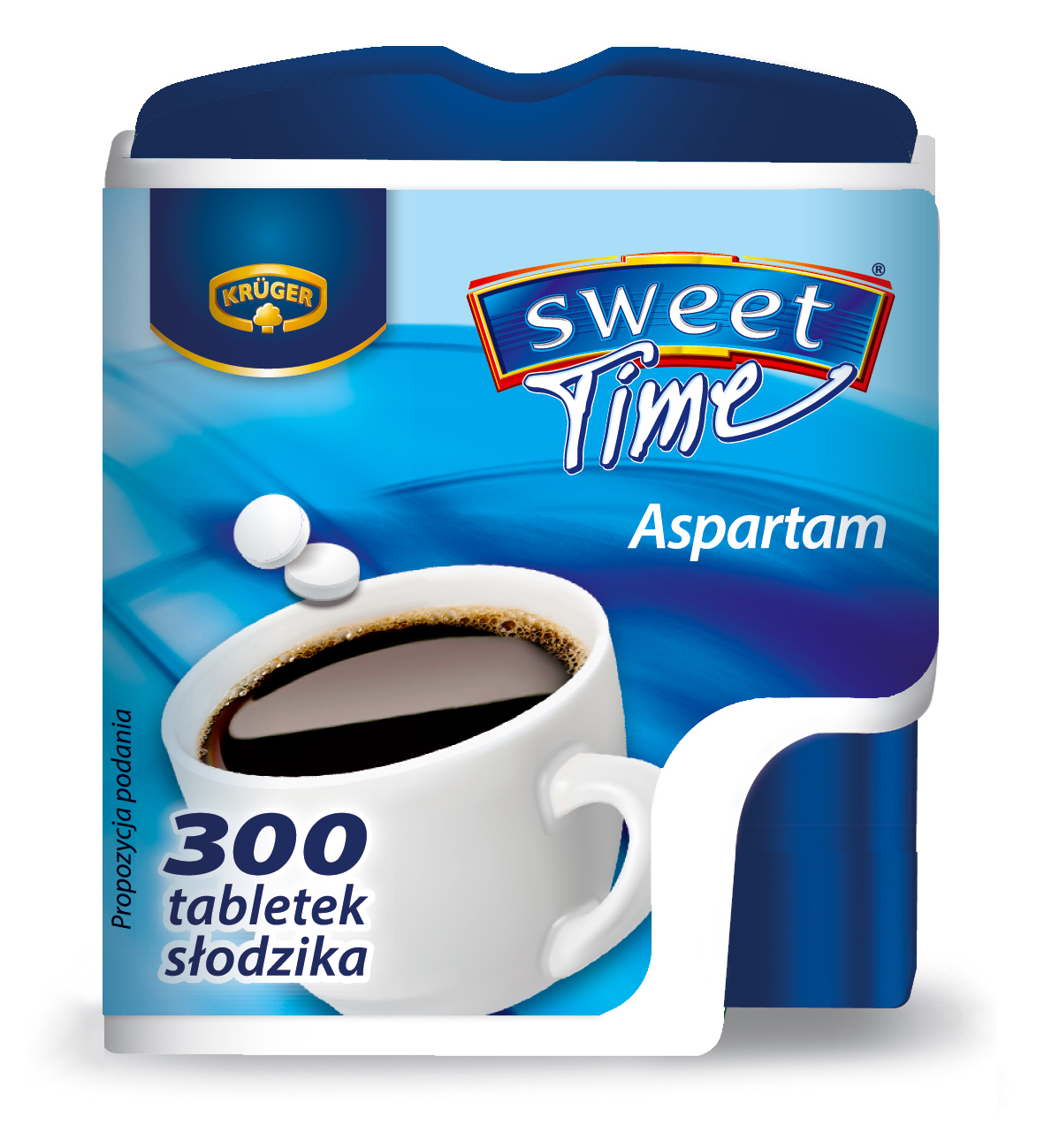The image depicts an illustration of a product packaging for an artificial sweetener, specifically aspartame, housed within a blue-lidded, plastic container. Dominating the visual is a large coffee cup with two small, white tablets poised to drop into the coffee. The brand name "Kruger" is prominently displayed in the upper right corner, along with the product name "Sweet Time Aspartam." Below the coffee cup, the text in what appears to be Polish reads "300 Tabletek Slodzika." The colors are predominantly dark blue, white, gold, yellow, various shades of blue, black, and brown, all balanced and evenly spread out within the design. Additionally, a distinctive blue button is featured at the top of the container, with an indented section in a darker hue located at the lower right, indicating where the tablets are dispensed. The style and composition clearly suggest this is a detailed illustration of product packaging rather than a photograph.